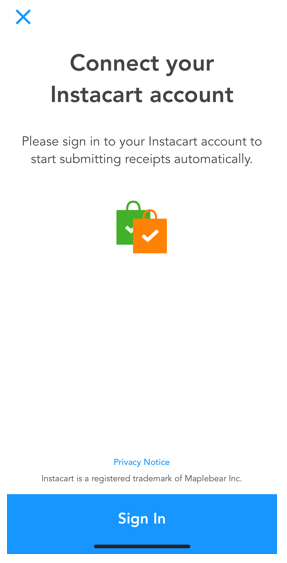This is a screenshot from a smartphone displaying the interface of an app or website prompting the user to connect their Instacart account. At the top-left corner, there is a small blue "X" icon. Below this, the phrase "Connect your Instacart account" is prominently featured in bold black letters, with the words "Connect" and "Instacart" both capitalized. The background is a clean, white color.

Just beneath the main title, there's an instruction in small gray lettering that reads, "Please sign into your Instacart account to start submitting receipts automatically." This provides guidance on what the user needs to do next.

In the center of the screen, there are two overlapping shopping bag icons. The bag in the back is green with a partial white check mark and a green handle. In front of it, there's an orange bag also bearing a white check mark, partially covering the back bag.

Following a large blank white space, towards the bottom of the screen, the phrase "Privacy Notice" appears in turquoise text, both words starting with capital letters. Below this, it reads, "Instacart is a registered trademark of Maple Bear Incorporated."

At the very bottom, there's a turquoise banner with the text "Sign In" in white, accompanied by a black underline marking the clickable button.